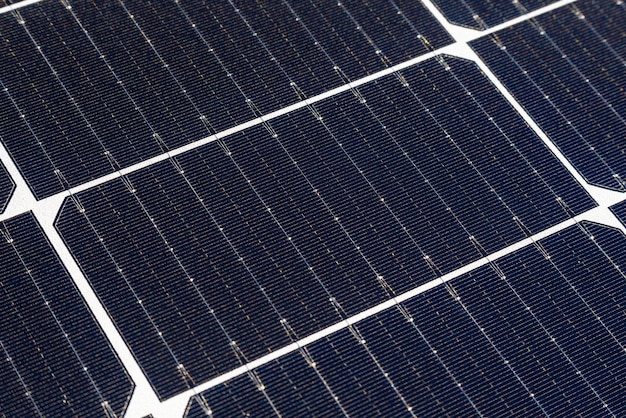The image appears to be a computer-generated close-up of a series of rectangular, blue-tinted panels arranged on a dark blue, grainy background, resembling an industrial or mechanical setup. Each panel is positioned at a 45-degree angle, with the bottom right and bottom left corners sharply defined, while the top right and top left corners are slightly truncated, forming a distinct geometric pattern. The panels are lined up in rows, partially overlapping, with the central panel fully visible and others extending beyond the edges of the image. 

Each rectangular panel features numerous fine, white vertical stripes running from top to bottom, segmented with small dots and seams, creating a tiled appearance. A notable feature is the chunkier white line that frames the borders of these panels, forming neat rectangles. Amidst the vertical lines, there are elements resembling electrical or mechanical connectors, with some lines appearing to end in fork-like prongs and others dotted with precise, evenly spaced markings. 

The panels are situated on a white surface, which enhances their blue hue and metallic silver plating, suggesting a high-tech or industrial application. The surfaces of the panels appear to be glassy, with hints of wiring interspersed, adding to the mechanical aesthetic. Overall, the composition is densely packed, emphasizing the interconnected nature of the panels, which might be part of a larger, sophisticated system.